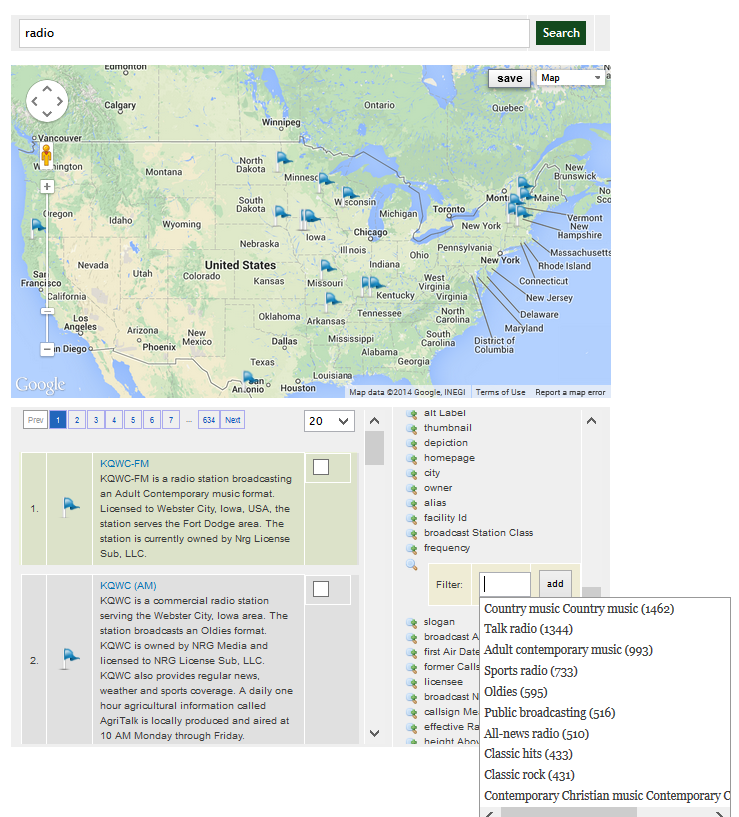**Detailed Caption: Map of Radio Stations Across the United States**

This image is a screenshot of a web page showcasing a map of the United States, prominently displayed in the upper portion. At the top of the page, there's a search box where the term "radio" has been entered. Adjacent to the search box on the right is a green search button. The map is dotted with several blue flag pins indicating the locations of radio stations.

Below the map, detailed descriptions correspond to each blue flag pin placed on the map. The first entry, labeled as number one, describes **KQWC-FM**: a radio station broadcasting an adult contemporary music format, licensed to Webster City, Iowa, USA. This station serves the Fort Dodge area and is currently owned by NRG Licensed Sub LLC.

The second entry, labeled as number two, details **KQWC-AM**: a commercial radio station also serving the Webster City, Iowa area. This station broadcasts an oldies format and is similarly owned by NRG Media and licensed to NRG Licensed Sub LLC.

In the right panel of the lower part of the webpage, there is a filter option for refining search results. A drop-down menu is visible because someone has clicked inside the filter field. The drop-down menu lists various filter options for radio stations, including categories such as country music, talk radio, adult contemporary, sports radio, oldies, public broadcasting, classic rock, and contemporary Christian music, among several other options.